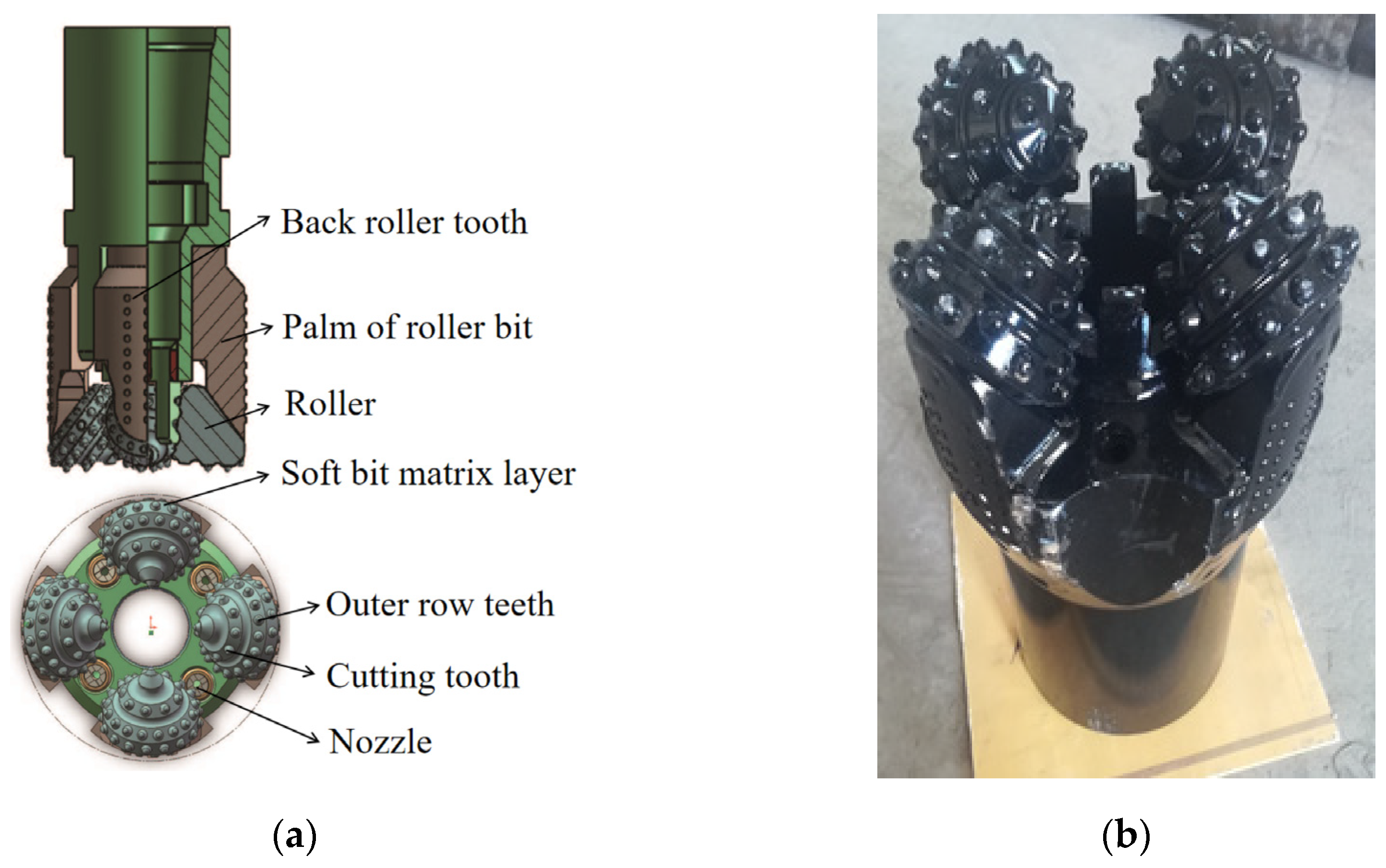The image depicts a heavy-duty, industrial drill bit designed for penetrating tough materials, characterized by its dark, spiked surface to provide traction as it digs. It is mounted on a yellowish rug, creating a stark contrast. The left side of the image features a detailed, hand-drawn plan of the tool, marked 'A,' with labeled components such as the back roller tooth, palm of the roller bit, roller soft bit matrix layer, outer row teeth, cutting tooth, and nozzle—all pointing to specific parts on the tool. To the right, a digital photograph marked 'B' showcases the actual drill bit in three dimensions, revealing more intricate details like a copper-colored steel drum base sitting on what appears to be white or stainless steel. Call-outs from the drawing correspond directly to the parts in the image, providing a comprehensive look at both the schematic and real-life structure of the equipment.